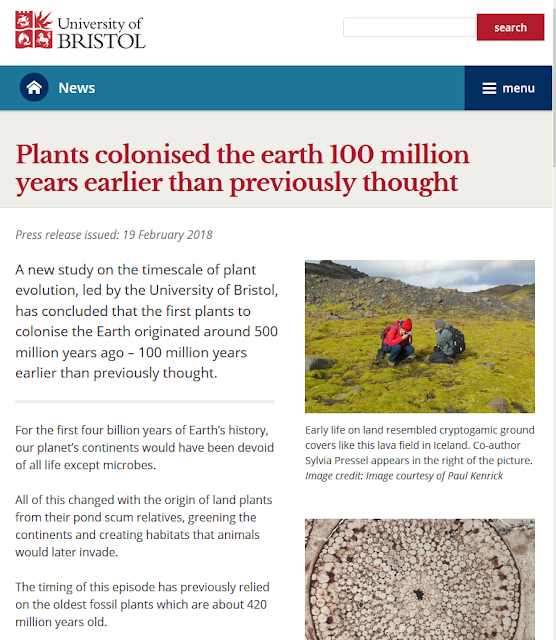Screenshot from a web device, likely a tablet, depicting a University of Bristol press release page with their coat of arms logo in the top left corner. The interface includes a search bar in the top right, a home button labeled "Home," a "News" section, and a "Menu" option represented by three horizontal lines on the far right. The headline in red text on a gray bar reads: "Plants colonized the earth 100 million years earlier than previously thought." 

On the far right, a thin scroll bar is visible. The press release, dated 19 February 2018, features two images. The first image shows two individuals standing in a rocky field with peat moss surrounding them. The second, located beneath the first, appears to be an enhanced microscopic image of plant life. The story discusses a University of Bristol-led study on plant evolution, revealing that the first plants colonized Earth around 500 million years ago, which is 100 million years earlier than previously assumed. Co-author Sylvia Pressel is visible in the right part of the field image. The study suggests early terrestrial life resembled cryptogamic ground covers similar to those found in a lava field in Iceland.